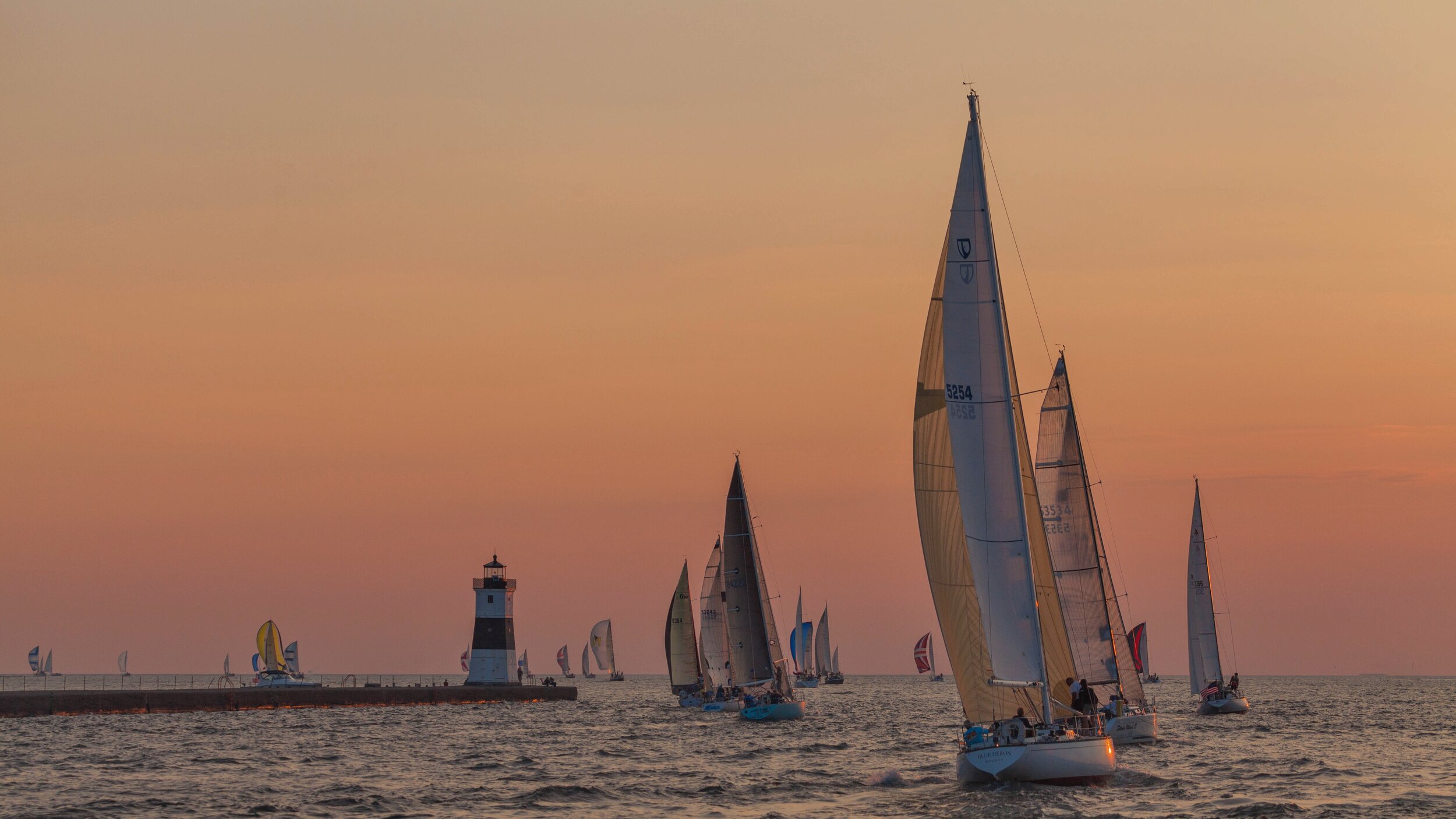This photograph captures a picturesque seaside scene dominated by a vast, pastel-colored sky transitioning from pinkish and yellowish hues into blue. The setting sun casts a dim, ethereal light over the multitude of sailboats navigating the ocean. Over a dozen sailboats populate the image, growing progressively smaller as they recede into the distance. In the foreground, the most prominent sailboat features a striking large yellow sail with a white middle portion, while other sails display shades of blue, red, and gray. The water beneath them appears as a deep, dull gray, reflecting the moody sky above. A notable architectural feature is a lighthouse situated along a pier extending from the left side of the image. This lighthouse stands as a sentinel over the sea, adding a touch of human presence to the serene natural tableau.